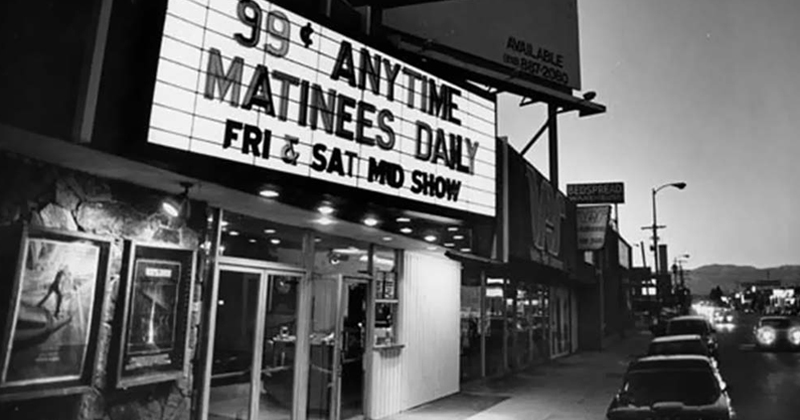The black and white photograph depicts a small, vintage movie theater likely set in the 1950s. The theater’s marquee, illuminated and prominently displayed, advertises "99 cent anytime matinees daily, Friday and Saturday MD show." In front of the theater are glass entrance doors flanked by poster displays within glass cases on a stone wall. The scene is set at dusk or in the early evening, evident from the cars with their headlights on parked and driving along the street to the right. The theater is part of an old-time strip mall with adjacent storefronts, though most signage is illegible except for a distant "bedspread" sign and a blank billboard with the number 887-2080. The ambient details include visible streetlights against the skyline, which are not yet illuminated.